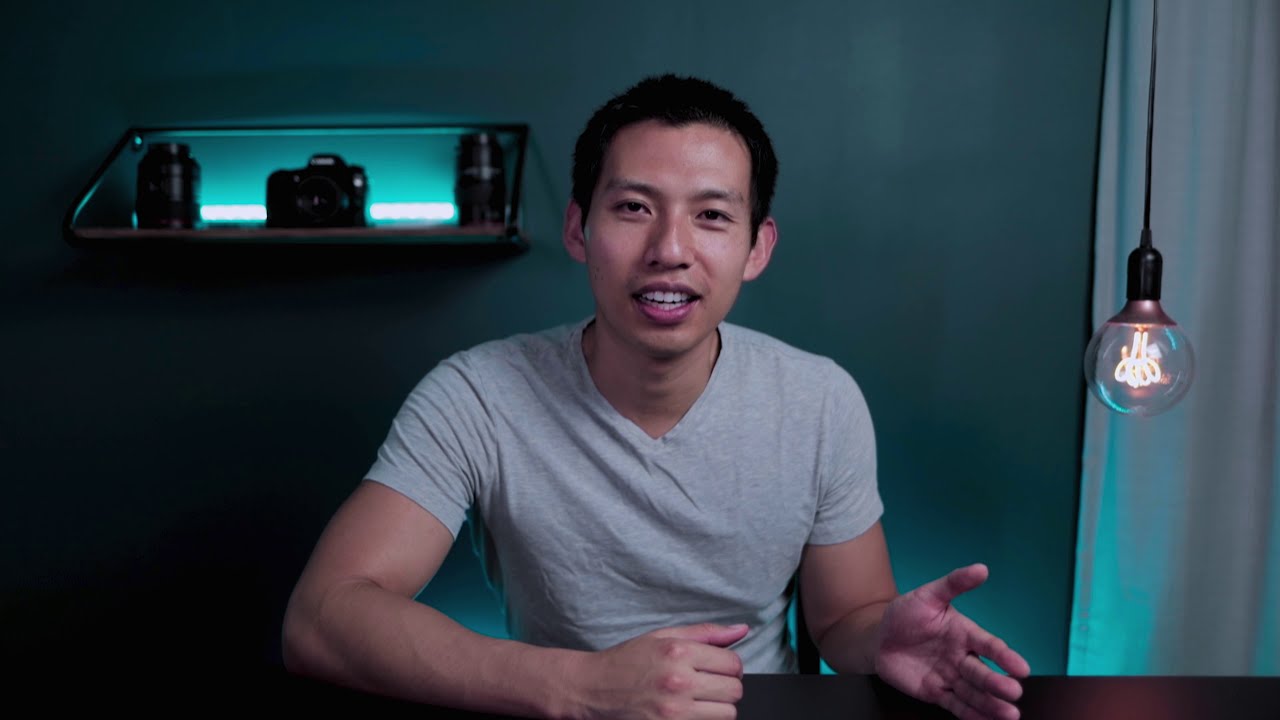This is a detailed landscape photograph of a young Asian man, likely in his 20s or early 30s, sitting in a dimly lit room. He has short cropped black hair and is wearing a light gray v-neck t-shirt. He appears to be speaking or mid-conversation, with his mouth open, and is gesticulating with his hands: his left hand is open with the palm facing towards the camera, while his right forearm rests on a wooden table, closed into a fist. 

In the background, the wall is dark green or turquoise, and there's an illuminated shelf displaying three items, including a camera and two lenses, bathed in a soft teal light. To the right of the man, a single wire hangs from the ceiling, suspending a round, clear light bulb with a lit filament and a black base, approximately two feet above the table. A light drapery is partially visible behind the light fixture. The scene is devoid of any text or additional objects, emphasizing the intimate, focused ambiance.